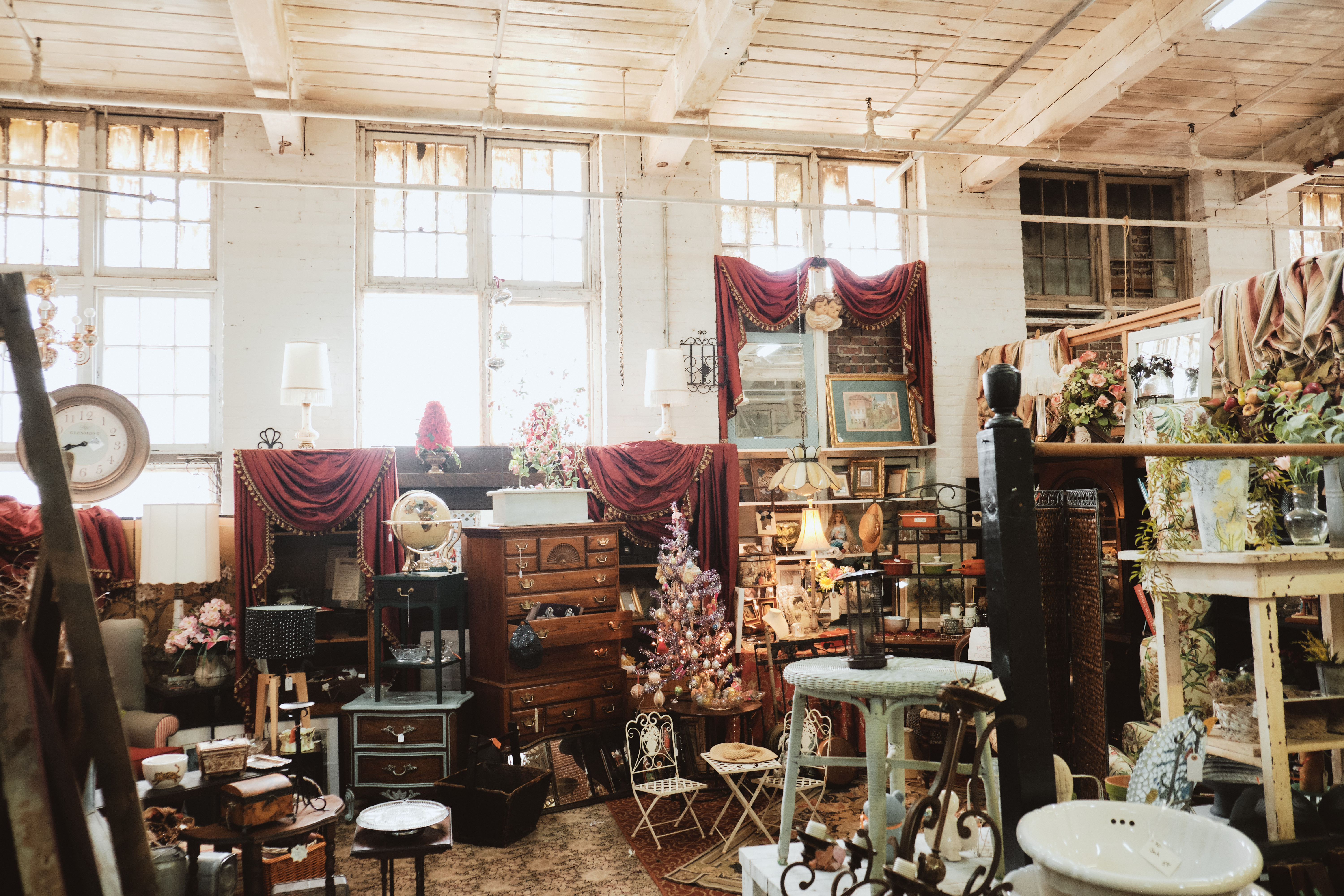The image depicts the cavernous interior of a very cluttered antique store. The space is filled with an eclectic assortment of collectibles and vintage items. Dominating the background are three large multi-pane windows with red draped curtains, letting in natural light that creates a bit of glare. The walls are painted white and the ceiling is unfinished, exposing wooden beams and rafters. The wooden floor is partially covered with various rugs.

The room overflows with items: a small white Christmas tree stands amidst the chaos, surrounded by wicker wastebaskets, foldable chairs, and children’s wire furniture including a small table and chairs set. There are numerous shelves packed with fake plants and a dresser with one drawer open. A table with an hourglass sits beside another table that has a stand topped with a globe.

On the left, an old clock and a large bookcase housing framed pictures, knickknacks, and vases of flowers add to the clutter. Jewelry cases and various boxes are stacked atop one another. The foreground features a slightly out-of-focus brown metal framework. This room is a treasure trove of antiques and curios, each piece vying for attention amidst the organized chaos.